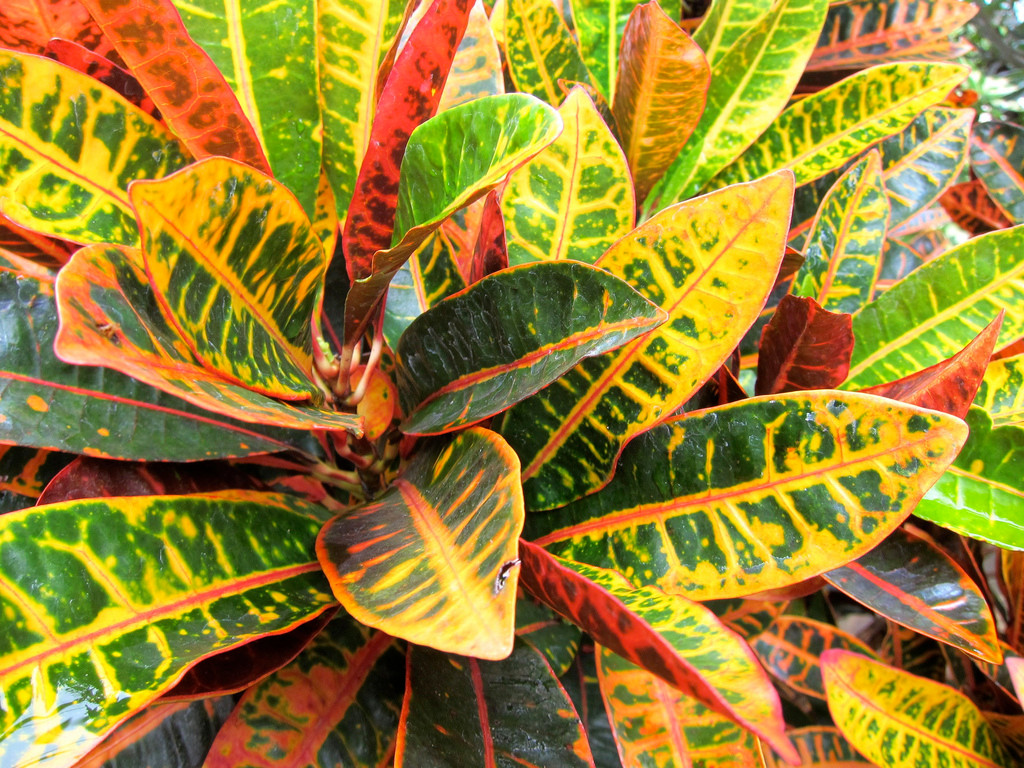The image showcases a vibrant, leafy plant occupying the entire frame. The leaves display a rich palette of colors, including green, yellow, orange, and dark green with striking red spines and veins. Some leaves have intricate patterns with yellow speckles and horizontal stripes, while others feature orange and red edges and splotches. The foliage appears to come from a central stem, extending outward in all directions, creating a lush, dense cluster that fills the image. The large leaves, adorned with red veins running vertically through their spines, suggest a natural setting rather than a potted house plant. The overall effect is a mesmerizing tapestry of color and texture.